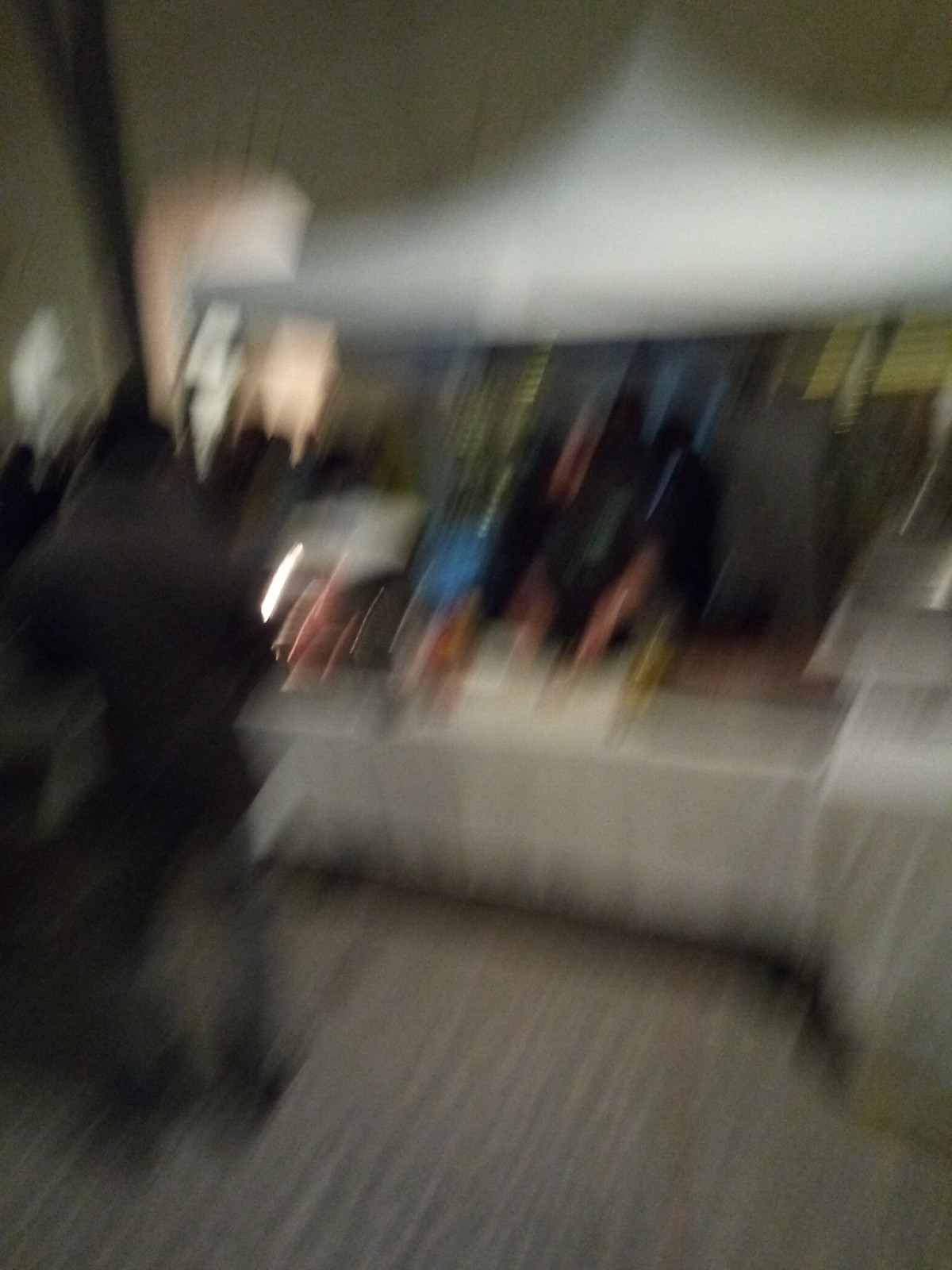The image is noticeably blurry and of low resolution, making it difficult to discern specific details. Despite the poor quality, the image seems to depict a scene with at least two people. On the left side, there is a discernible outline of a person, visible from the legs upward. In front of this person, there is a long, white counter. Behind the counter stands another individual, whose hands can be faintly seen resting on the surface. The scene appears to be set under a white roof tent, adding context to the environment despite the overall fuzziness and lack of clarity.